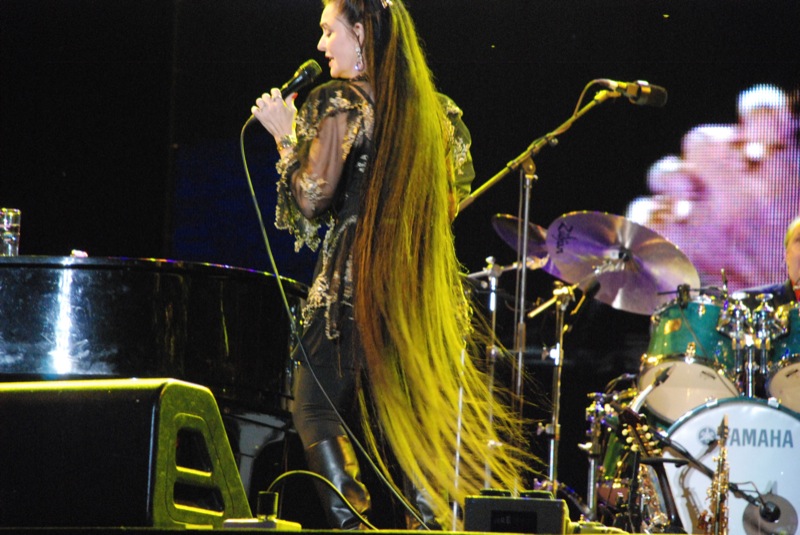In the photograph, a Caucasian woman with extremely long, straight brunette hair, streaked with blonde highlights and brushed by green stage lights, stands at the center of an intensely lit stage, her eyes closed as she passionately sings into a black microphone. Her back is turned slightly towards the camera, obscuring her outfit, but you can make out a sheer black blouse with gold trim, paired with black pants and ankle-high black leather boots. The background is a deep, solid black, shrouding the environment and leaving the focus solely on her performance.

Surrounding her on stage is an array of musical instruments: a green and white drum set to the right, accompanied by a slightly visible older white male drummer, a gold-colored saxophone and a black acoustic guitar both resting on stands in front of the drum kit. To her left is the edge of a grand black piano, its shiny surface catching the stage lights. In the bottom left corner, a large black speaker is partially cropped by the frame, angled towards the singer. The contrast between the singer's illuminated figure and the dark, indistinct surroundings creates a captivating and dramatic scene, encapsulating the essence and energy of the concert.